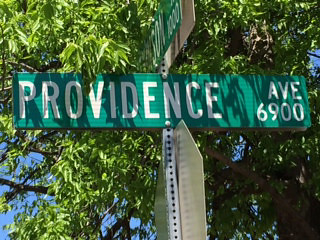In this small photograph, we see the backside of a standard octagonal stop sign, mounted on a roughly one-inch square metal post that is perforated with holes. Above the stop sign, a green street sign reads "Providence Ave 6900." Perpendicular to this street, another street sign (partially obscured) seems to indicate a name ending with “S-O-N” and a number, likely “1,000.” The background features lush vegetation, including a large tree with green leaves, and a portion of clear blue sky is visible.